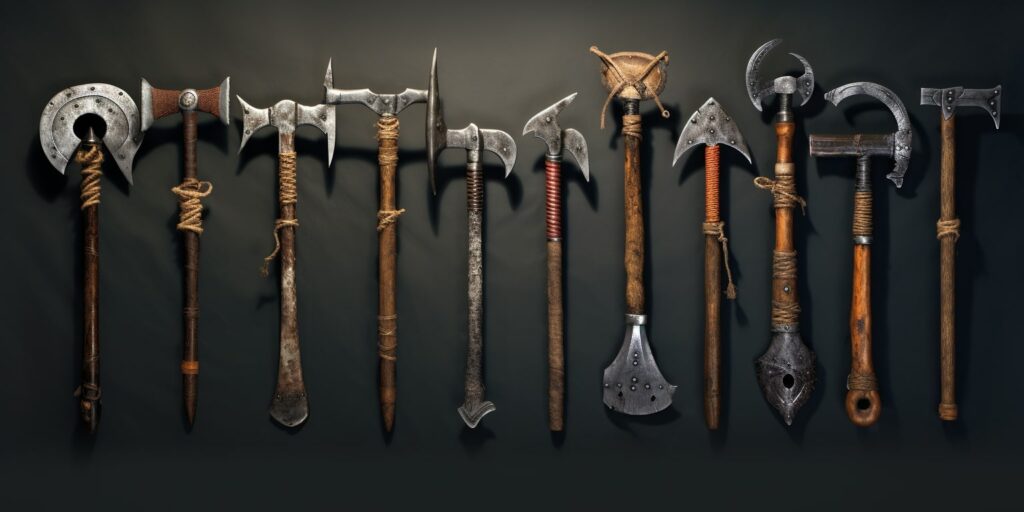The image is a rectangular landscape, approximately twice as wide as it is tall, featuring a black wall backdrop that is illuminated by a light source at the top center. Displayed on this wall are 11 various handheld weapons, primarily axes and hatchets, arranged vertically with their heads mostly at the top, except for the seventh weapon, which is pointed downward. The weapons appear weathered and old, with an authentic look, suggesting they might be modeled after ancient or medieval tools likely from the Viking era. Some weapons feature intricate designs, including double-edged axes, spiked blades, and possibly even spade-like implements. The handles, mostly wooden and wrapped in twine or rope near the blades, exhibit distress and signs of aging, contributing to their antique appearance. The heads of these weapons are primarily made of distressed metal, possibly steel or copper, and exhibit variations such as rounded edges, deep points, and curved-down blades, adding to the diversity and historical intrigue of the display.